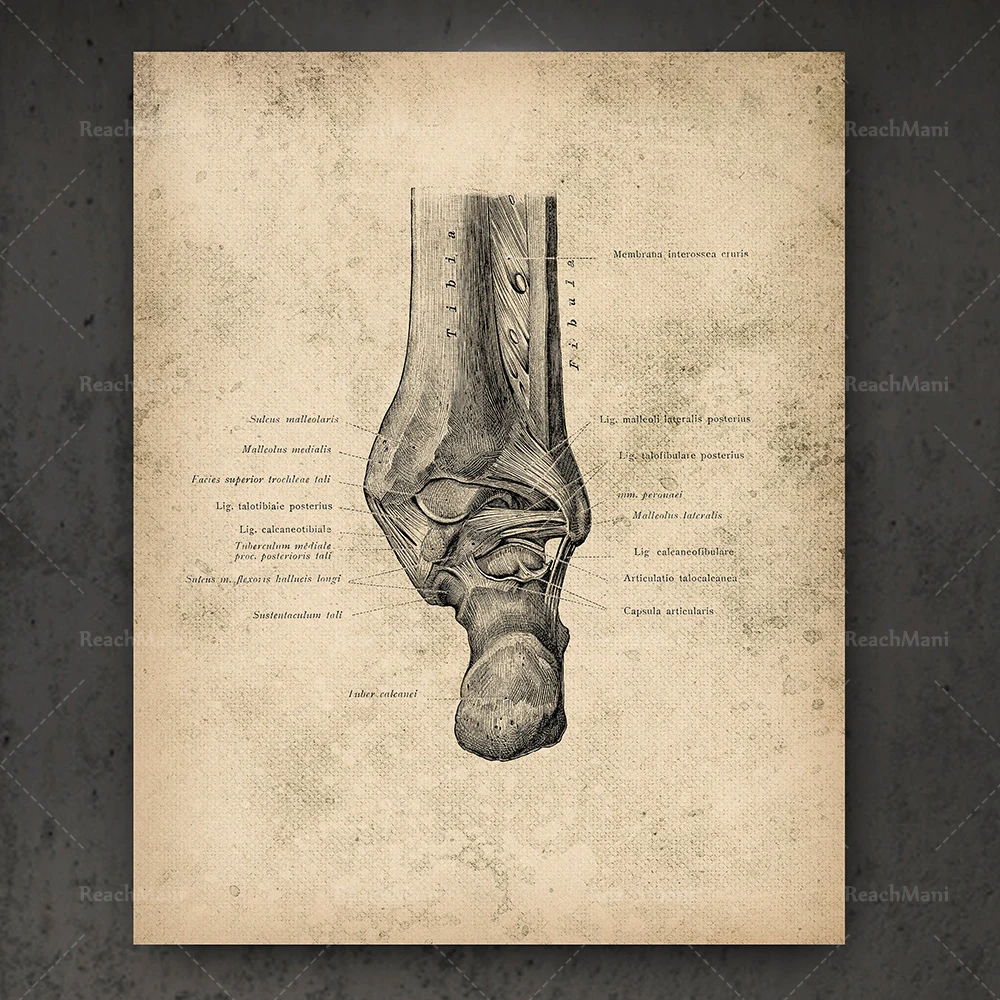This detailed, black-and-white antique medical drawing meticulously illustrates a human lower leg, focusing on the tibia and fibula bones, along with their associated joints and muscle areas. The well-documented diagram includes numerous labels for parts such as the sulcus malleolus and malleolus medialis, offering a comprehensive anatomical guide. The parchment, aged and faintly stained, suggests the use of traditional drawing implements like charcoal, adding to its intricate shading and detail. Additionally, the document carries a watermark of repeating crosses and currency symbols, signifying its protection against unauthorized use. The overall appearance hints at the image originating from an old, well-used medical book.